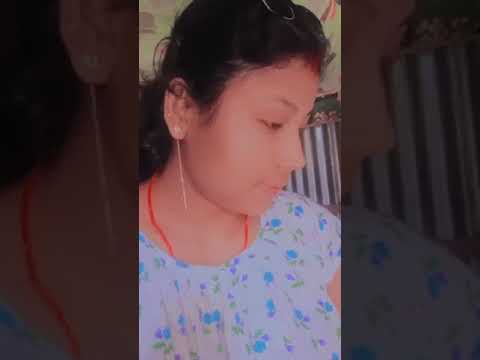This photograph, captured with a cell phone camera, predominantly features a young woman who appears to be in her 20s, with medium light to brown skin and dark brown or black hair pulled back into a ponytail. She is adorned with a single earring on her right ear, which dangles about five inches, and a delicate red beaded necklace that complements her attire. Her blouse is white, decorated with a floral pattern in shades of blue, green, and purple. The woman is captured in profile, gazing downward to her left with a neutral expression, characterized by downcast eyes and a straight-lipped mouth. The photograph itself occupies the central third of the image, while the left and right thirds are darkened and enlarged portions of the same image, adding a sense of depth and focus on her serene figure. Background details include some indistinct wall hangings and a lattice frame behind her.